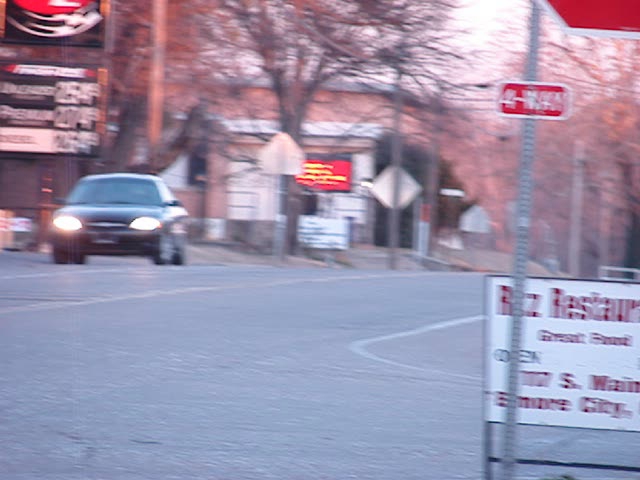This is a color photograph taken outdoors during the daytime, capturing a slightly out-of-focus small-town intersection scene. The top right corner of the image features a partially visible stop sign with the word "four-way" written in white on a red background, indicating an all-way stop intersection. Below the stop sign, a restaurant sign, partially obscured by the stop sign pole, seems to say "Ritz" and mentions its location as South Main, Elmore City, along with an "open" notice in red text on a white background. The left side of the photo includes a gas station with a clearly visible blue car exiting, headlights on. The gas prices, though blurry, appear to be $2.54 for unleaded and $2.74 for premium. The surroundings include tree-lined streets without leaves, suggesting a fall setting, and small buildings typical of a small town, including various business signs. Several road signs such as stop and yield signs are visible but facing away from the viewer. The overall scene is marked by blurred movement, likely due to camera motion.